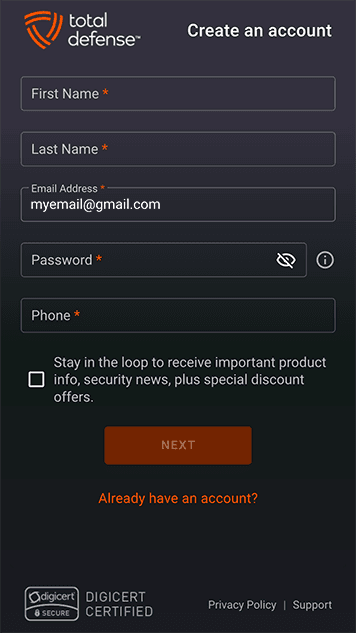The image depicts a sign-up page for "Total Defense," an online service or application. Situated at the top left corner, the Total Defense name is accompanied by its logo, which is a badge-like emblem in orange. Directly to the right of the logo, the phrase "Create an Account" is prominently displayed in white.

The form below includes several input fields that prospective users must complete:
1. **First Name** - Marked with a red asterisk indicating a required field.
2. **Last Name** - Also indicated with a red asterisk for mandatory information.
3. **Email Address** - The placeholder text within the box suggests using an example format such as "myemail@gmail.com."
4. **Password** - Accompanied by a red asterisk, this field also features a crossed-out eye icon, suggesting password visibility control. Additionally, there is an "i" (information) icon for further guidance.
5. **Phone Number** - Required as indicated by the accompanying red asterisk.

Below these fields, there is a checkbox option with the label: "Stay in the loop to receive important product info, security updates, plus special offers." 

At the bottom of the form, an orange button with the word "Next" in white lettering invites users to proceed to the next step of the sign-up process.